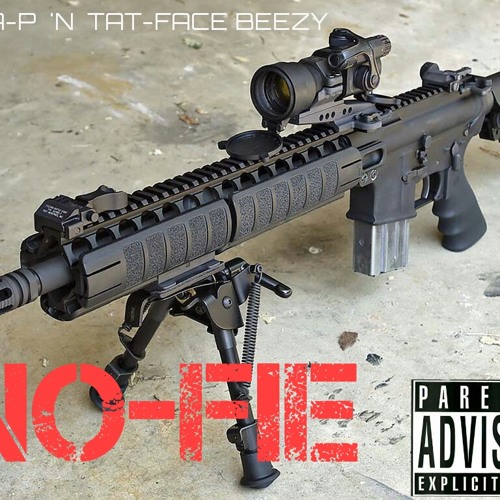This image features a black, automatic rifle equipped with a prominent cooling jacket and mounted on a two-legged tripod, suggesting it's designed for stability and sustained use. The gun chamber appears substantial, potentially indicating that it's loaded. Atop the rifle sits a detailed viewfinder with a mini telescopic appearance, complete with a flip-up front cover to protect the lens. Additionally, the firearm includes a handle and a clip, contributing to its practical functionality. The rifle is positioned on a cement ground, devoid of any visible human presence or time markers.

Text is inscribed on the image, notably in the top left corner with the words "A-P-N-T-A-T-F-A-C-E-B-E-E-Z-Y," which may refer to a name or model designation. The text at the bottom appears fragmented, showing partial letters like "O-F-I-E." Additionally, the phrase "Parental Advisory Explicit" is discernible in the lower right corner, suggesting a logo or warning. Another text snippet, "PARAY, ADVIS, NO FEE," is present but its meaning remains unclear, possibly indicating it's in another language.